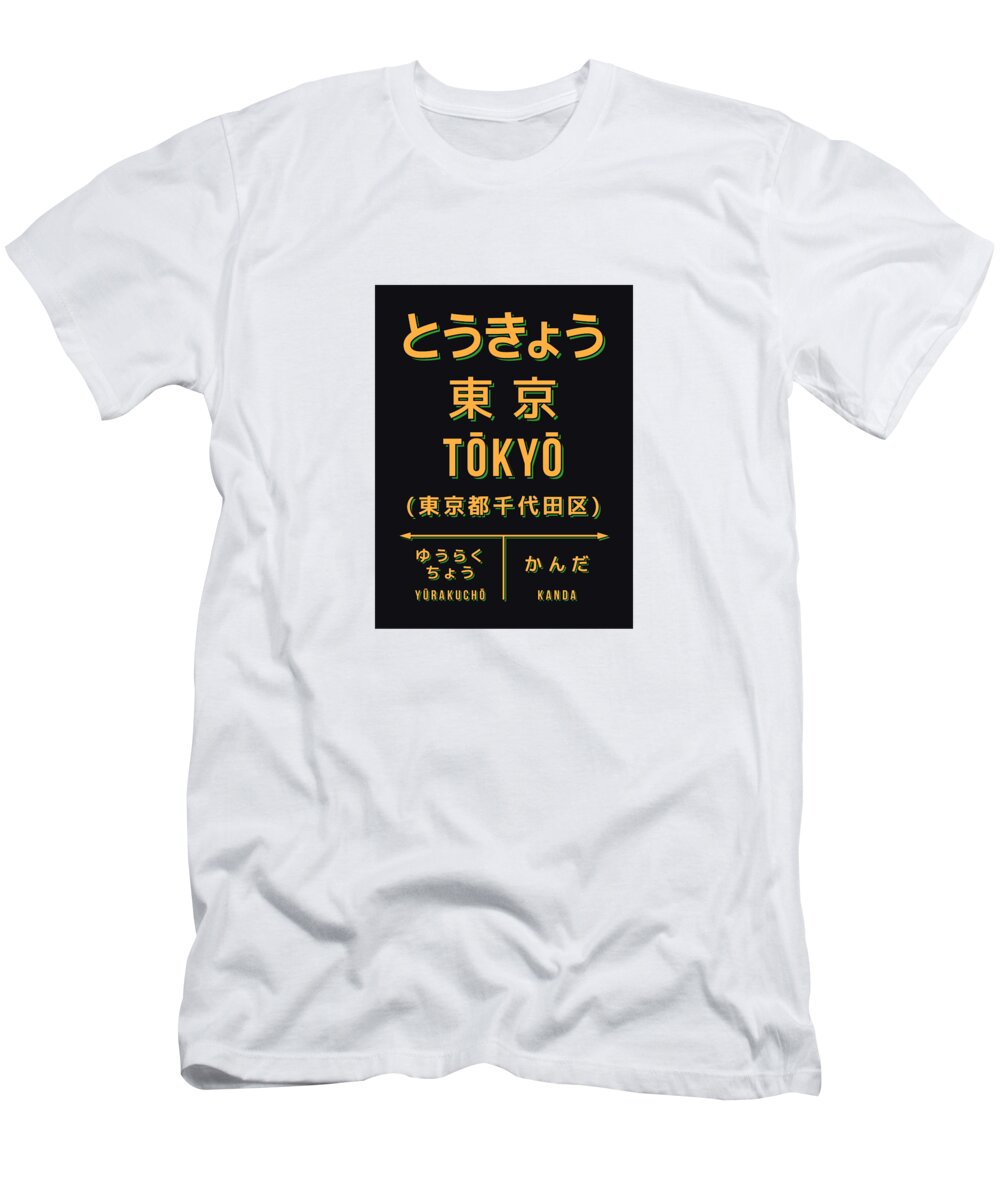This is a detailed description of a white, short-sleeved, crewneck t-shirt. The focal point of the shirt is a prominent black square situated in the center. Within this black square, yellow lettering features prominently. The first two rows of the text consist of Japanese characters, followed by the word "Tokyo" in the third row, and "Tokyo" again in the fourth row. Below these, there appear to be additional sections, with arrows pointing left and right from a central line, also in yellow, giving the impression of a design meant to convey directional information or event details.

Further text on the shirt includes "Yorikucho" and "Kanda," which are presented alongside more Japanese symbols. These names are likely referencing specific districts or locations within Tokyo. The shirt itself is quite clean, devoid of any visible stains, but it does exhibit several wrinkles, suggesting it may have been recently folded or moved. The edges are trimmed, and despite the wrinkles, the shirt maintains a neatly pressed appearance. The overall design is stylish, with a blend of cultural elements and modern aesthetics, reminiscent of a concert series t-shirt.